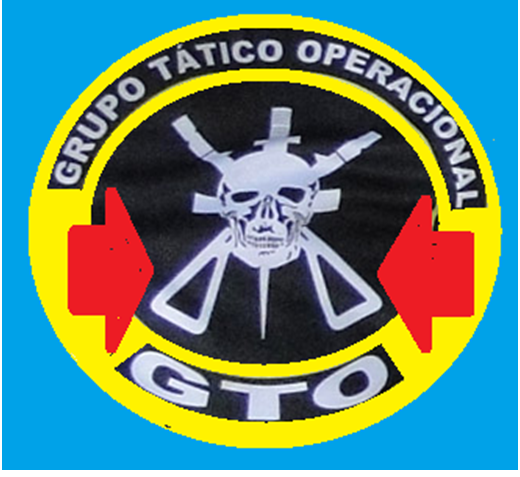The image features a striking emblem positioned against a solid bright blue background, resembling an organizational patch. At its core is a black circle displaying a prominent white skull. Flanking the skull are pairs of white triangles extending outwards from either side. Red arrows on each side point inward toward the triangles, adding to the design's dynamic feel. This emblem is set within a larger yellow circle with an enclosing band at the top containing text in Spanish that reads "Grupo Tactico Operacional," suggestive of a Tactical Group Operations unit. Below the black disc, another black band bears the bold white letters "GTO."